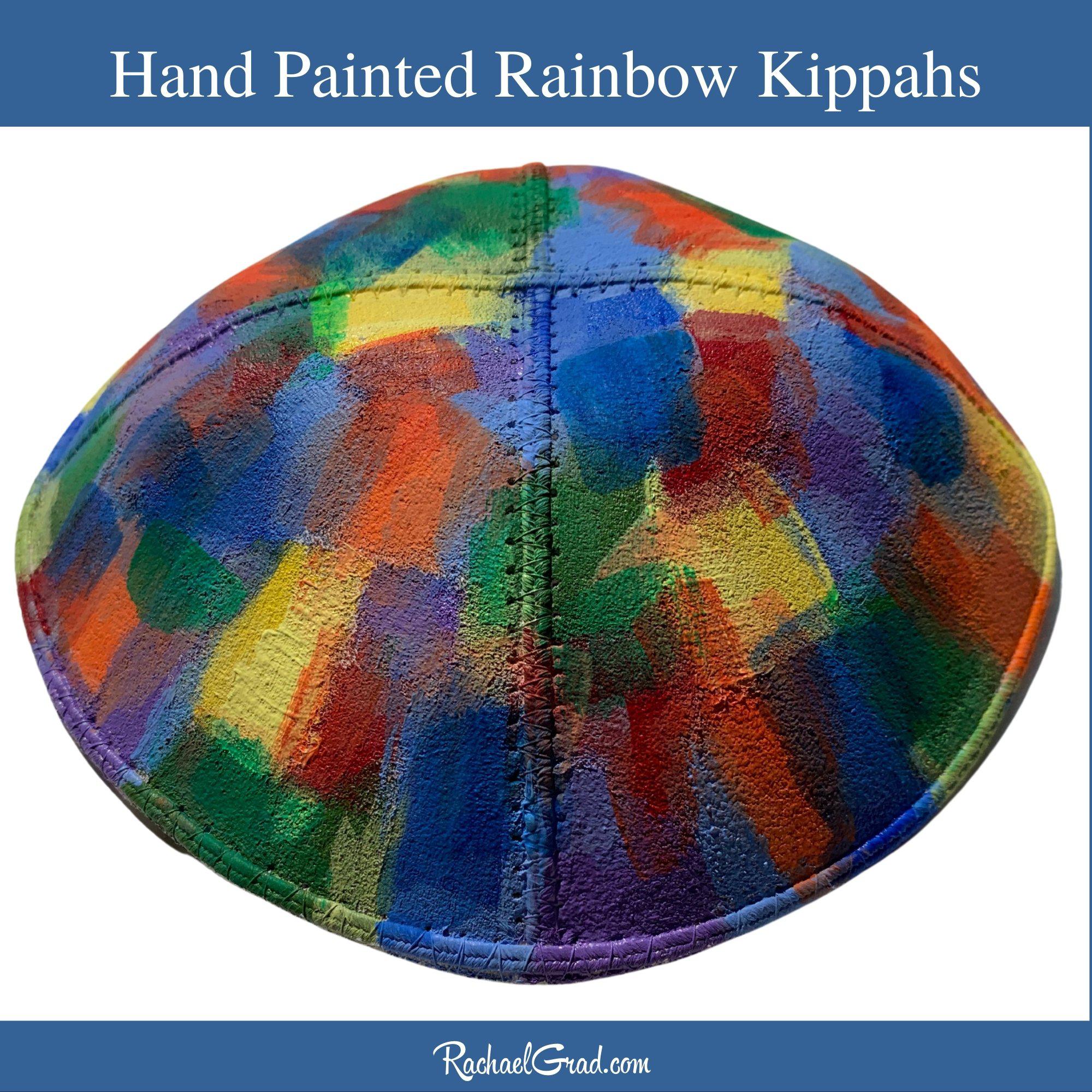The image features a hand-painted rainbow kippah, prominently displayed on a completely white background. The kippah consists of four triangular panels sewn together, creating a cross pattern at the top, and has a stitched brim all around. The panels are adorned with vibrant brushstrokes in a range of colors, including red, orange, yellow, green, blue, and purple, lending the kippah a distinct, multi-colored, impressionist aesthetic. At the top of the image, white text on a blue background proclaims, "Hand-painted Rainbow Kippahs," while the bottom of the image features the text "RachelGrad.com," indicating the creator or vendor. The entire design showcases an artistic and painterly approach, highlighting the unique, hand-crafted nature of the kippah.